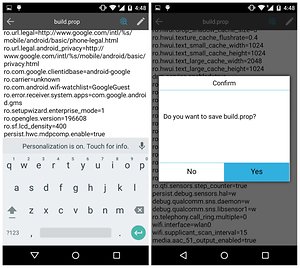The image consists of two screenshots from the website build.prep. 

The screenshot on the left features a white window filled with rows of text, likely relating to coding. At the bottom of this window is a virtual QWERTY keyboard with a black header and footer. The keyboard displays a line above it stating, "Personalization is on, touch for info," along with a microphone icon on the far right. Key features include a numbers button on the bottom left, a space bar in the center, and a teal arrow button pointing to the right on the bottom right.

The screenshot on the right shows another section of the build.prep website. The background is grayed out, and a white pop-up window appears in front. The pop-up window is titled "Confirm" at the top and contains the message, "Do you want to save build.prep?" At the bottom of this message are two buttons: a white "No" button on the left and a blue "Yes" button on the right.